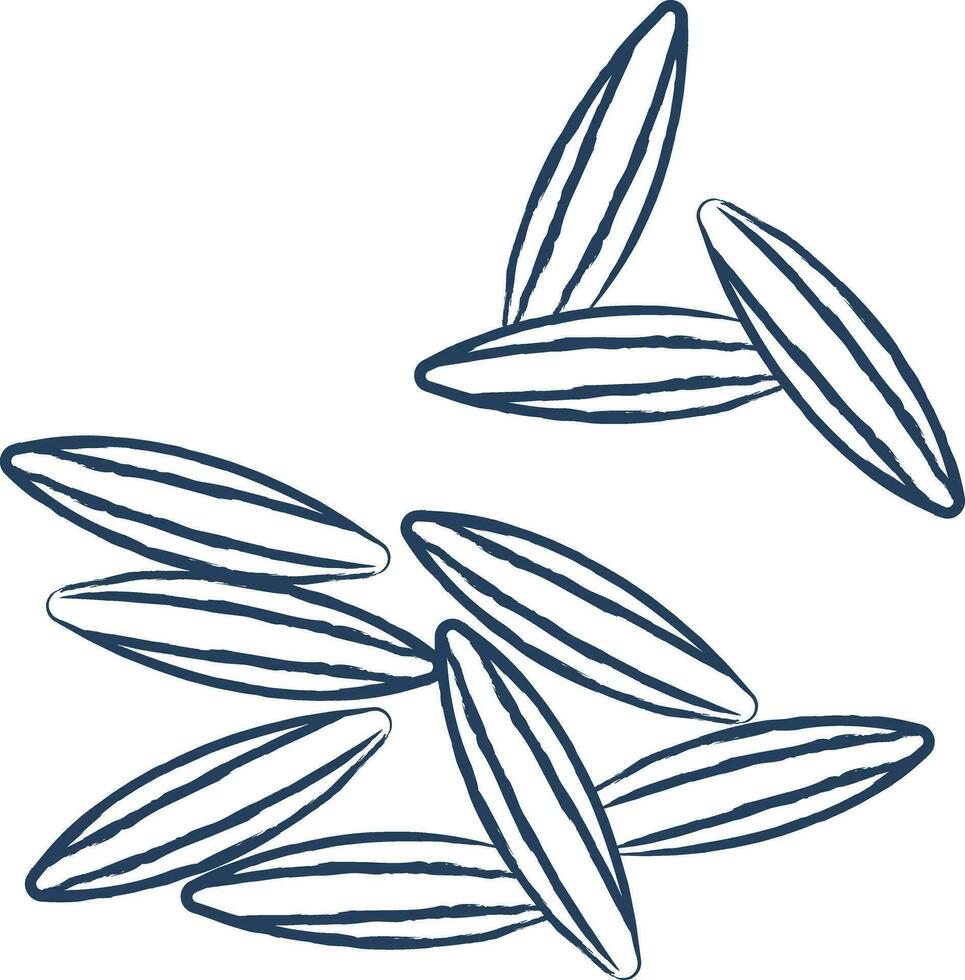The image depicts a simple, computer-generated array of 10 elongated, sharply pointed ovals, resembling seeds or cucumbers, on a white background. Rendered in a dark blue or greenish-blue color, each shape features two lines running lengthwise through the center, enhancing their resemblance to narrow seeds. The ovals are dispersed with a concentration of seven toward the bottom and three closer to the top. Their orientations vary, with some lying horizontally, others diagonally, and one oriented vertically. The ovals appear to float in empty space, with no accompanying text, borders, or additional elements.